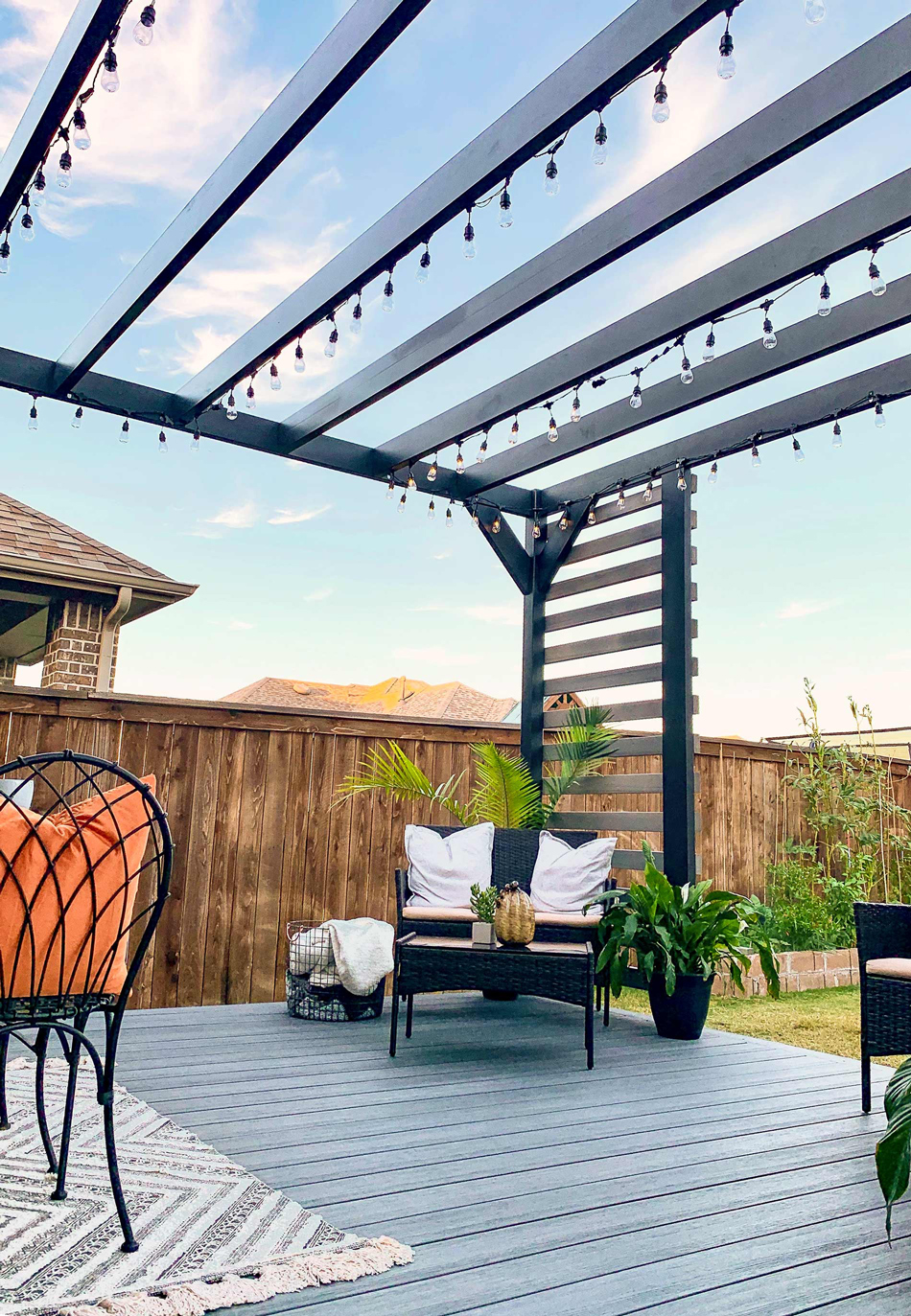The photograph, taken on a bright sunny day with a partly cloudy sky, captures a serene outdoor patio scene. The vertical image prominently features a transparent wooden pergola casting shadows on the deck below. Sprinkled with clear hanging light bulbs, the pergola adds a warm, inviting touch to the space. The deck is constructed from wooden slats and hosts a variety of comfortable seating arrangements including a black wicker chair with two large white cushions and a matching wicker table. There's also a black chair with an orange cushion, providing a splash of color. 

A black and white zigzag rug lies on part of the deck, upon which metal wire chairs are positioned. Potted plants, including ferns with large leaves, are placed around the deck, adding a touch of greenery. On one side of the deck, near a wicker chair, there’s a table decorated with plants in big pots and decor items. A wooden fence borders the yard, and beyond it stands a brick house with a visible downspout from the gutter. The yard itself features green grass and a garden filled with plants exhibiting tall stems and leaves. In the distance, a small mountain is visible, peeking above the fence, completing the picturesque scene.